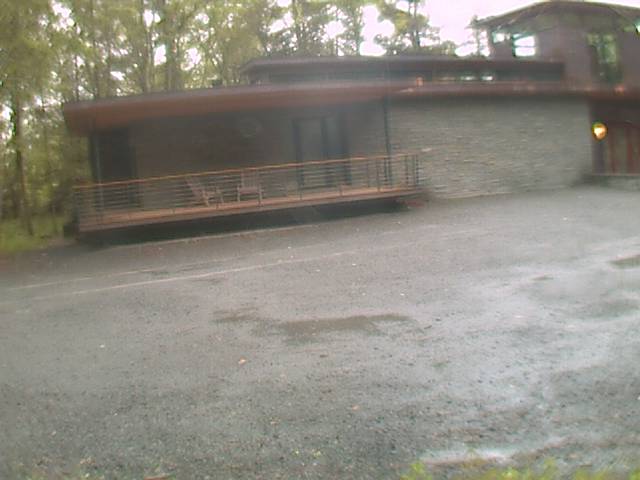This photograph captures a mid-20th-century, Frank Lloyd Wright-inspired stone house characterized by multiple levels and extensive use of natural materials. The lower level is constructed from limestone-like brick, while the upper floor features contrasting red brick. The scene radiates a serene, earthy ambiance with an abundance of browns in the house's design and wooden exterior elements. 

To the left, there is a spacious porch adorned with wooden Adirondack chairs and surrounded by a slightly reddish metal railing. Below the porch, the foreground consists of a gray, cement-like driveway with patches of wet asphalt and tiny pebbles, suggesting recent rainfall. The driveway stretches broadly in front of the house, possibly indicating a single-family residence despite its expansive size. 

There's a visible entranceway to the right with a light fixture or a reflective metallic circle near the door. The house sits in front of a dense wooded area with tall green trees creating a picturesque backdrop. The second story includes a distinct, almost tower-like structure, contributing to the home's unique and timeless architectural style.